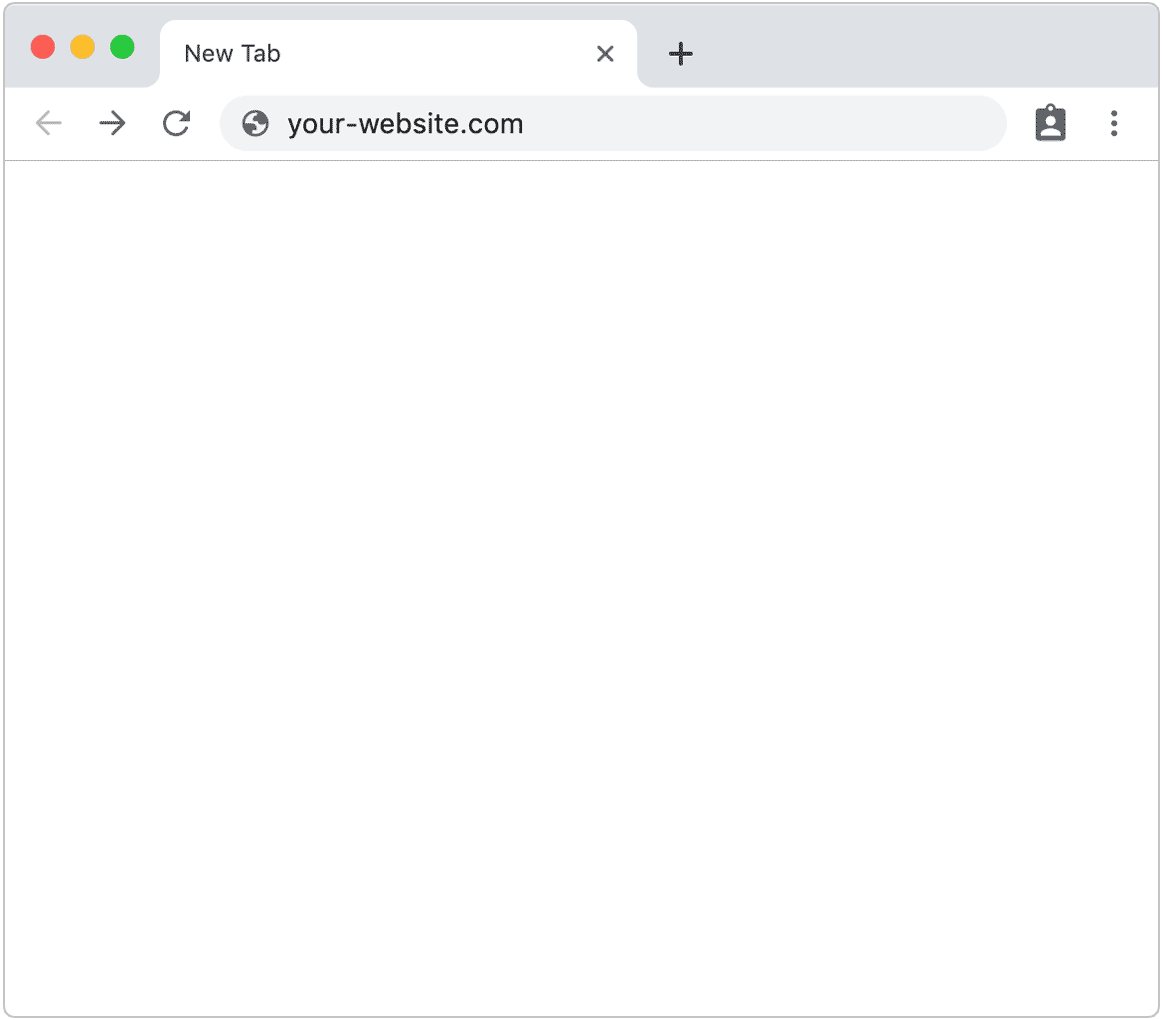This image features an internet browser window. The majority of the screen is blank, displaying an empty white canvas. At the top of the window, running from the left to the right edge, is a gray bar. On the left side of the gray bar, there are three center-aligned circles: the leftmost circle is red, the middle circle is yellow, and the rightmost circle is green.

Adjacent to these circles, slightly to the right, is a browser tab labeled "New Tab," which is left-justified within the tab area. This tab also includes a close button. To the right of the tab, there is a black plus sign, indicating the option to open a new tab.

Below the gray bar is the web address bar, which features navigation buttons on its left. Starting from left to right, the buttons include a back arrow, a forward arrow, and a refresh icon. In the web address bar itself, the text "your-website.com" is displayed.